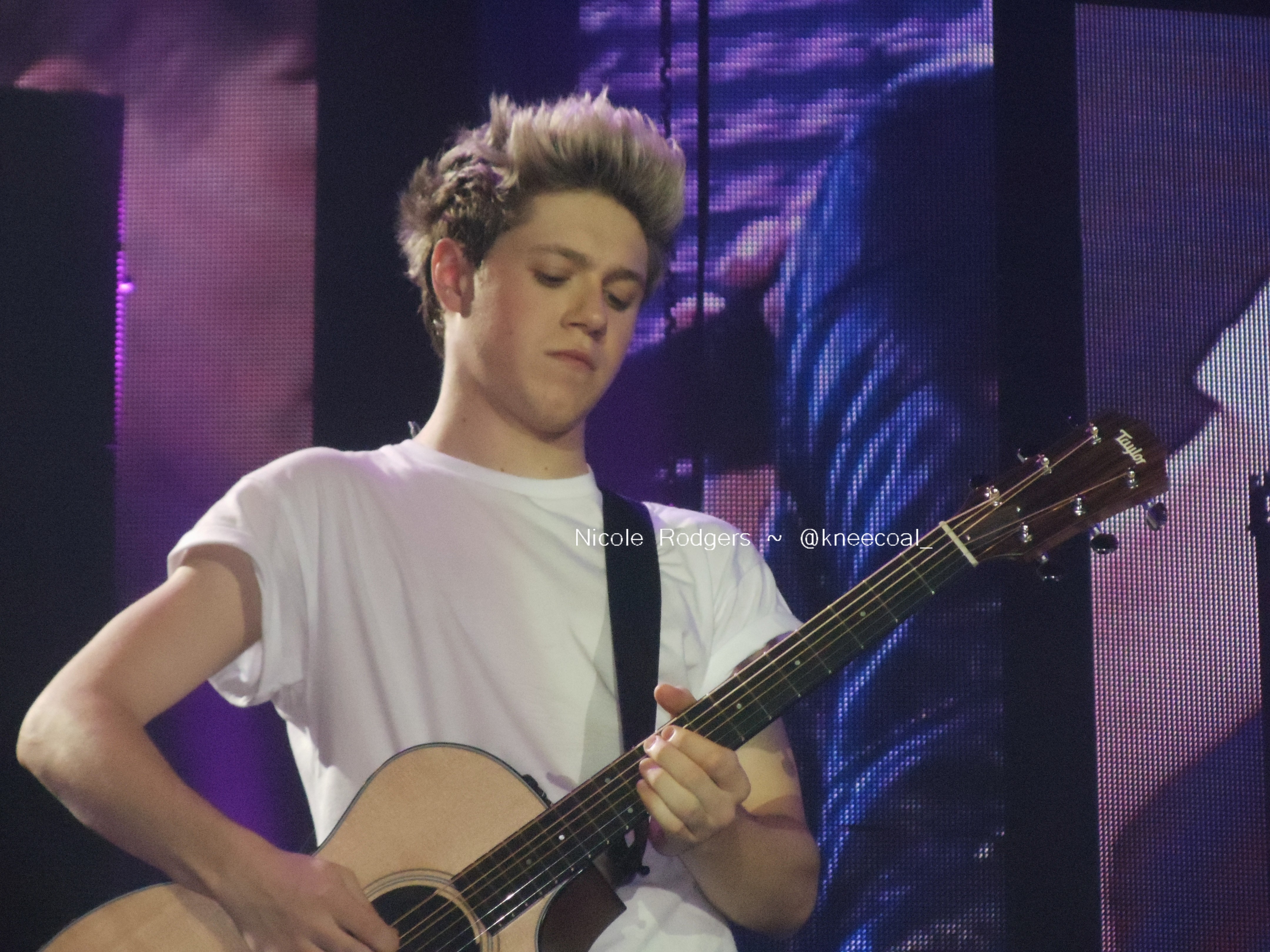This detailed photograph captures a young guitarist, likely in his late teens or early twenties, intensely focused on his acoustic guitar performance. He is positioned centrally, wearing a white t-shirt that highlights his skinny arms. His hair, blonde-brown and spiked around his ears, gives a dynamic look as if he could be headbanging. The stage where he performs features a large screen in the background displaying a bluish-purplish ambiance, enhancing the concert atmosphere. The young musician appears mid-action with his right hand strumming and left hand on the fretboard, deeply concentrated, possibly during a solo. The watermark "Nicole Rogers @Nicole" is visible on the image, subtly attributing the photographer. The overall scene shows a vibrant mix of colors including black, pink, purple, gray, blue, white, and tan, complementing the energetic setting of a live music event.